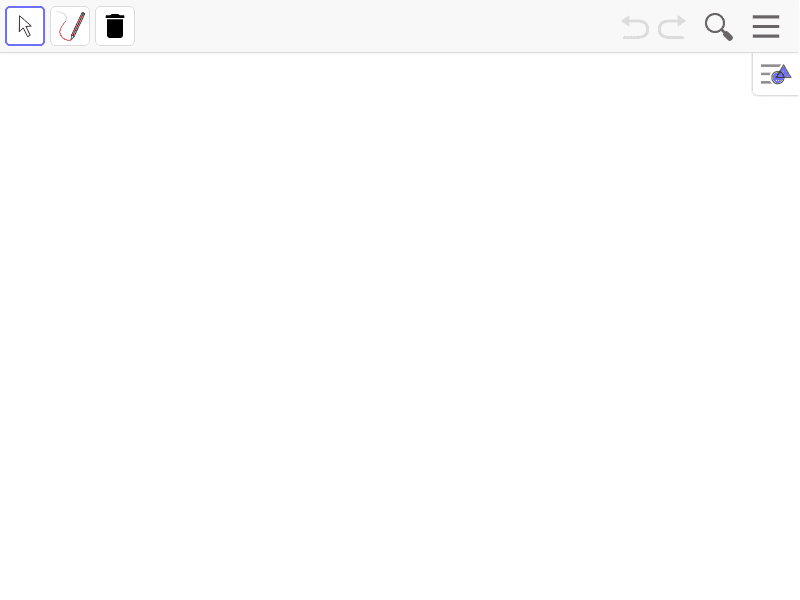The image is a small, detailed interface snapshot. 

In the upper left corner, the interface showcases two distinct rows. The first row has a gray background and contains three icons:

1. **Arrow Icon**: Located on the far left, this icon points to the upper left and is highlighted with a blue box, indicating it is currently selected.
2. **Pen Icon**: This icon resembles a pen that has drawn a squiggly line, suggesting it may be used for editing purposes.
3. **Trash Can Icon**: The final icon in this row is a black garbage can, likely used for deleting items.

Each icon is enclosed in a white box, with the exception of the selected arrow icon, which is enclosed in a blue box.

In the upper right corner of the interface, the row continues with:

1. **Gray Go Back Arrow**: A curvy arrow pointing left.
2. **Gray Go Forward Arrow**: A curvy arrow pointing right.
3. **Search Icon**: A dark gray magnifying glass.
4. **Menu Icon**: Three dark gray horizontal lines.

Directly below these icons, there is another image featuring three dark gray horizontal lines, but these are accompanied by a blue circle and a blue triangle, with the triangle positioned slightly above the lines. The entire secondary image is bordered by a white box.